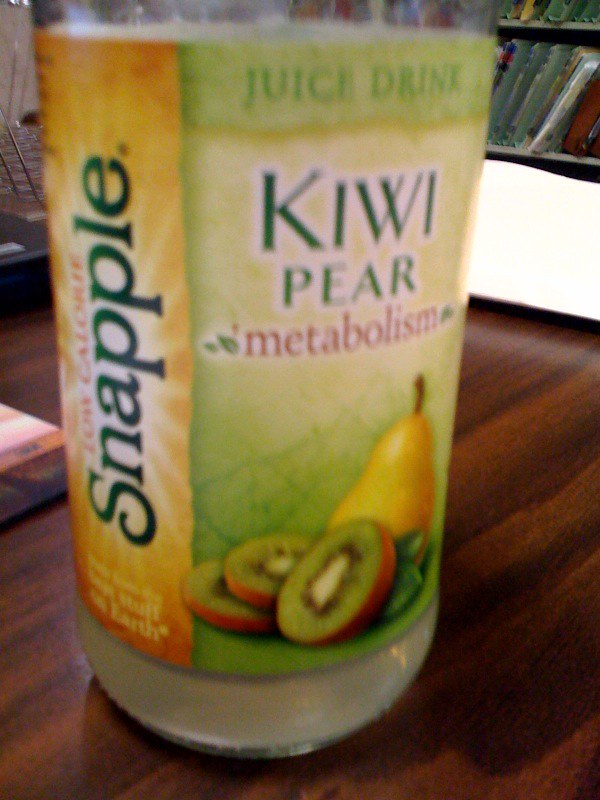On a wooden countertop, a laminated wood board is displayed centrally. To the upper right, a white sheet is partially visible. The shelf behind the counter is lined with numerous folders, each bearing colored labels in blue, red, yellow, and white. More folders protrude from the topmost shelf. On the far left, a set of metal bars can be seen. A paper is placed at the bottom. In the middle of the counter, there is a Snapple bottle. Leftmost is a Green Texas Snapple, followed by a Red Texas Low Calorie Snapple. A yellow rectangle is present in the backdrop. To the right, and positioned above, is a large Green Texas juice drink. Below it, there is a Kiwi Pear Snapple and a Red Texas Metabolism drink. The bottom of the scene features sliced kiwi and a yellow pear on the right.